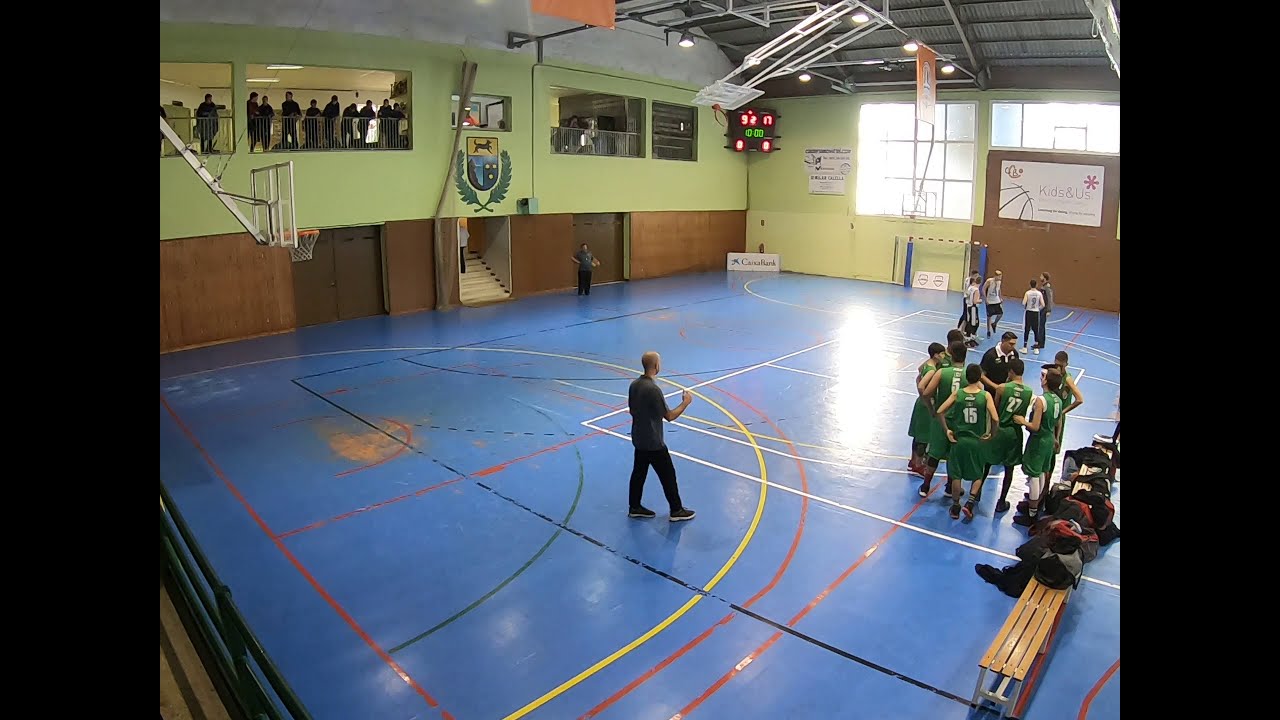This image shows an interior shot of what appears to be an old gym, likely part of a high school. The gym features a blue floor marked with red, yellow, green, and black lines, some of which are faded. In the foreground, a basketball team wearing matching green shirts and shorts is gathered around their coach, who seems to be giving them instructions. Visible jersey numbers include 5, 15, and 27. Another team dressed in white shirts and black shorts is grouped similarly with their coach nearby. Wooden paneling lines the lower half of the gym walls, while the upper part is painted light green, adorned with what seems to be the school's crest. Overlooking the scene, spectators are gathered behind a railing on the second floor. A scoreboard is located in the corner, completing the nostalgic atmosphere of the gym.